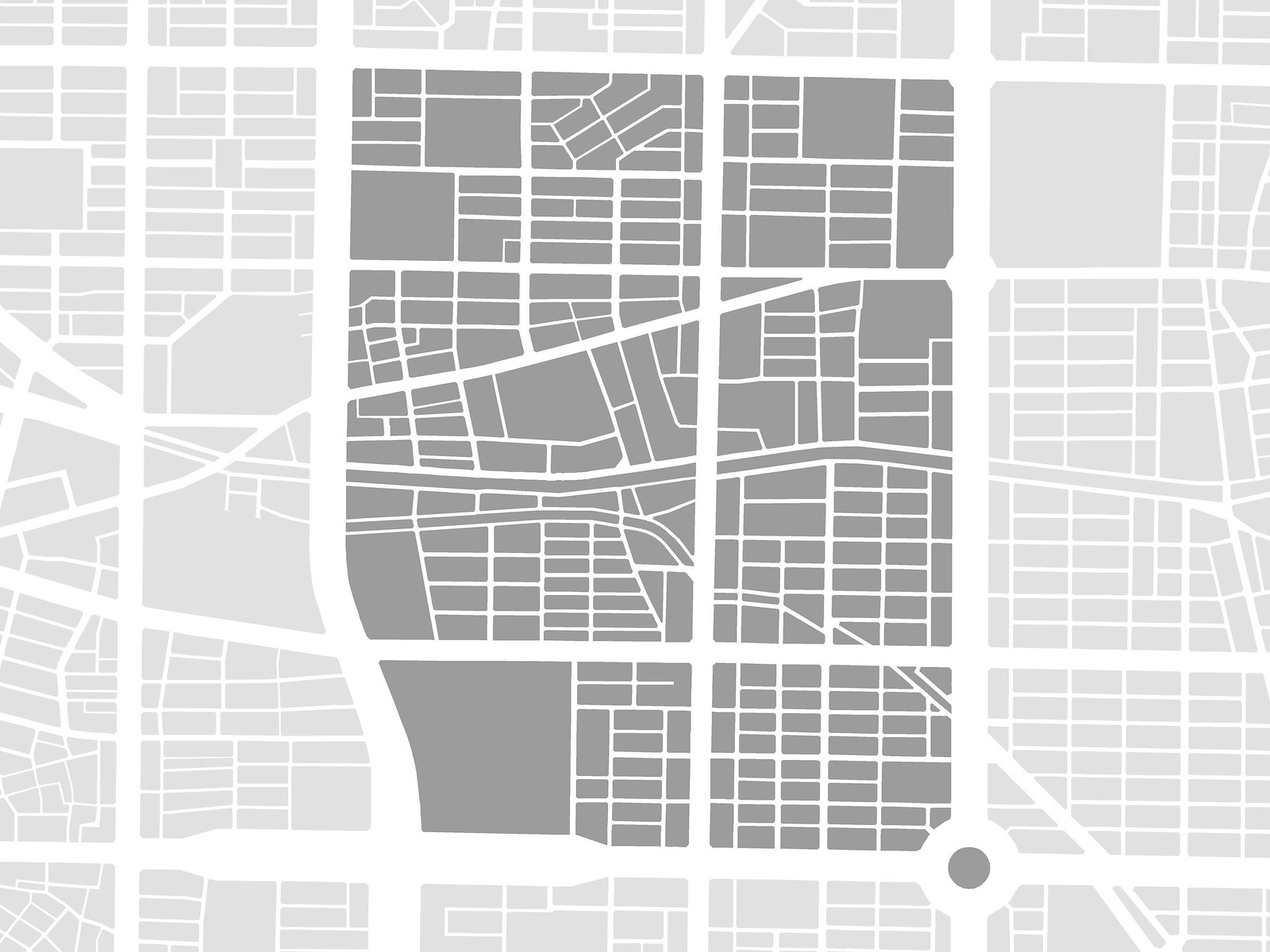The image depicts an unlabeled grayscale map focusing solely on the distribution of land sections and roads. Various shades of grey, including light gray, dark gray, and white, help differentiate between different areas and features.

The top of the image showcases a white road accompanied by seven neatly aligned segments above it. Directly below this, two light gray sections are visible, separated by a large vertically aligned road heading south. Adjacent to the large vertical road, there is a prominent gray section encompassing nine distinct subsections.

A large road extends further down toward the bottom of a dark gray area, which features a circular white traffic circle with a dark gray center. To the right of this traffic circle, four light gray sections can be observed.

On the left side of the map, a total of eight light gray sections are present. Some of these sections appear incomplete or partially outside the visible boundary of the image, providing an indication of the varying layouts. Each section includes numerous smaller divisions, with some lots appearing rectangular, others irregularly shaped, and some positioned at angles, while a few maintain a symmetrical pattern.

The overall map, lacking any labeling or water features, highlights the intricate layout of land divisions, emphasizing the structure and arrangement of lots within each section.